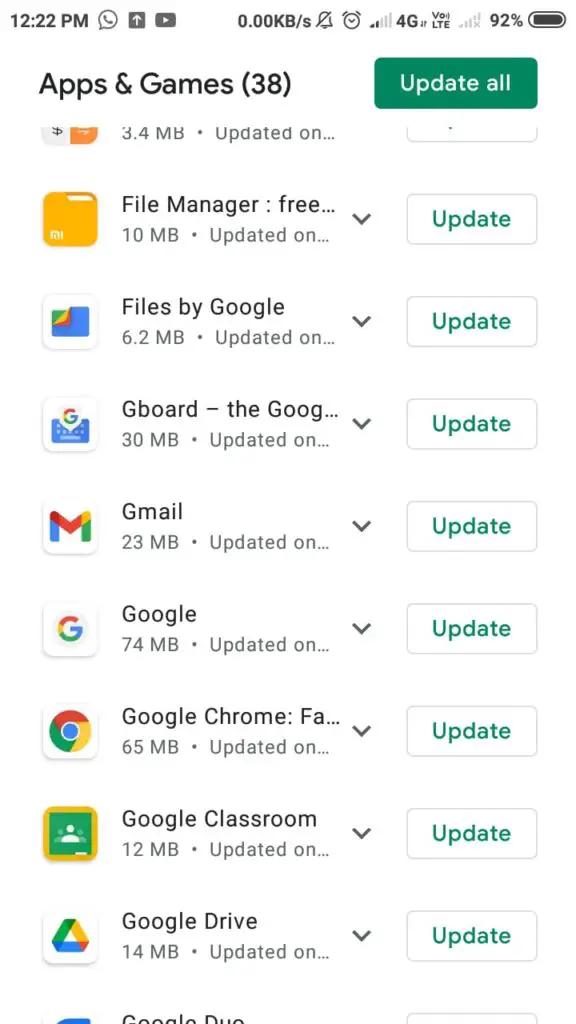In this screenshot of an Android device, the status bar at the top provides a wealth of information. At the top left, the device time is displayed as 12:22 PM. The status bar icons indicate current connectivity and notifications: there is a WiFi icon alongside a YouTube notification icon. Additional icons include a speed meter, a mute icon, an active alarm icon, and network signal bars for two SIM cards; SIM1 shows 2 out of 5 bars with 4G and voice over LTE, while the second SIM has no network signal. The battery level of the device is critically low, at less than 2%.

Below the status bar, a list of applications and their associated details is visible. The section titled "Apps and games" shows a total of 38 apps, with an option to update all. The file manager is consuming 10 MB, "Files by Google" is 6.2 MB, Gboard is 30 MB, Gmail is 23 MB, Google app is 7.4 MB, Google Chrome is 65 MB, Google Classroom is 12 MB, and Google Drive utilizes 14 MB.

The interface features a variety of colors, predominantly yellow, blue, red, green, and white, which visually differentiate entities and highlight important information.